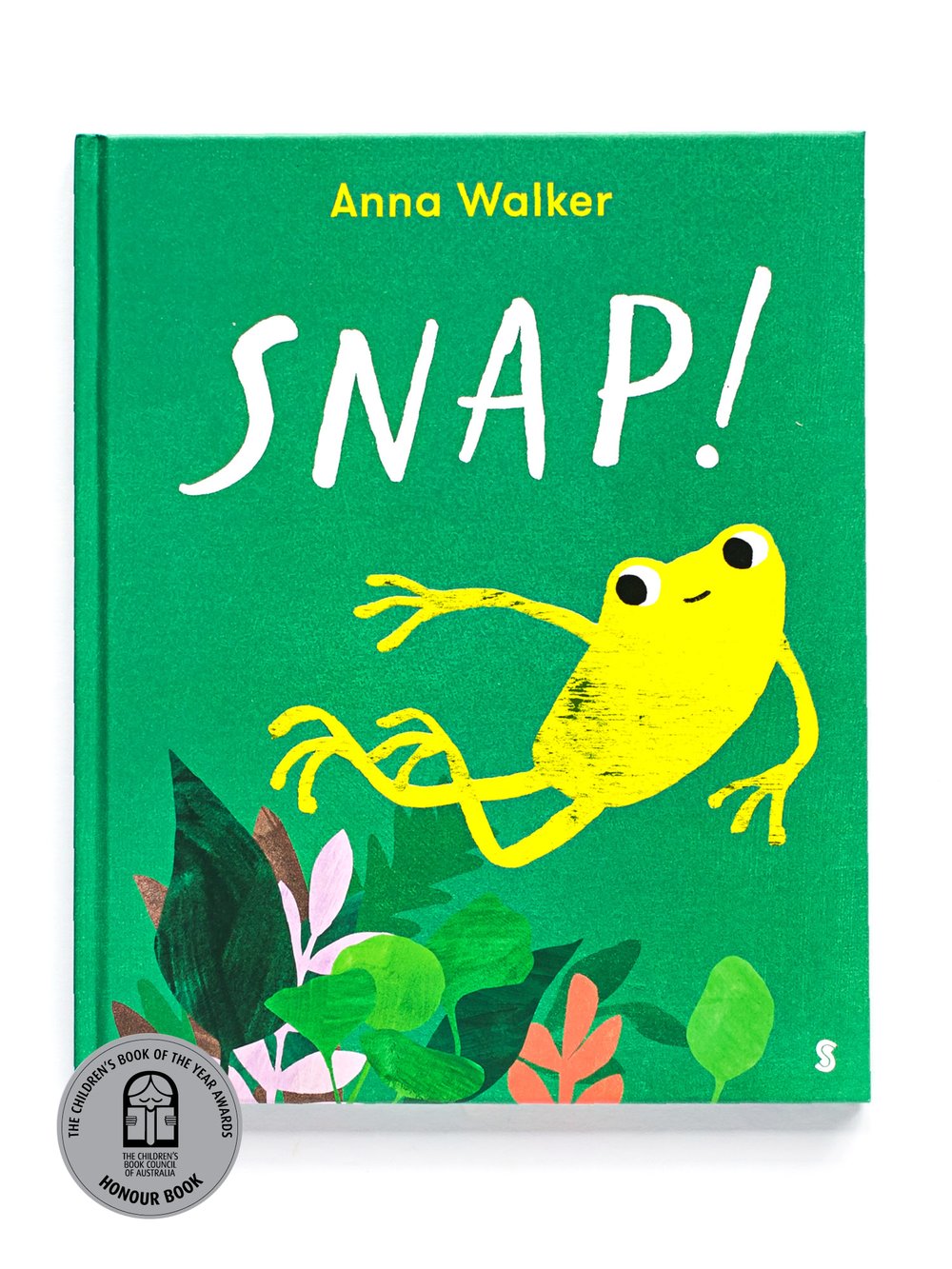This image showcases the cover of a vibrant green children's book titled "Snap!" by Anna Walker. The author's name, Anna Walker, is displayed prominently in yellow at the top, while the title "Snap!" is written in large, white capital letters followed by an exclamation mark. Below the title, a cheerful yellow frog with expressive black-and-white eyes is depicted leaping with loose limbs amidst an array of colorful foliage. The foliage includes various shades such as greens, pinks, browns, and possibly some coral hues, evoking a rainforest or wetland setting. At the bottom, a gray circular sticker denotes the book as an Honor Book in the Children's Book of the Year Awards by the Children's Book Council of Australia, featuring a small illustration of a person reading.